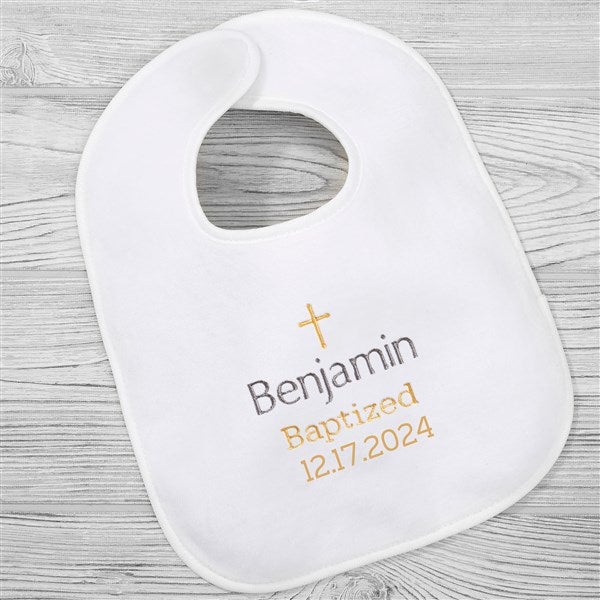This photo captures a white baby bib lying on a backdrop of a white and gray wood grain surface, which might be plank tile or a wooden table. The bib dominates the image, featuring solid white piping along its edges and a velcro fastener around the neck. Made from what appears to be a soft, terrycloth-like material, the bib is intricately embroidered. At the center, a golden cross is prominently stitched a couple of inches below the neck. Beneath the cross, the name "Benjamin" is embroidered in a dark gray or black thread. Further down, the word "baptized" is stitched in a similar gold thread, followed by the date "12-17-2024" in gold, almost in a Times New Roman font.